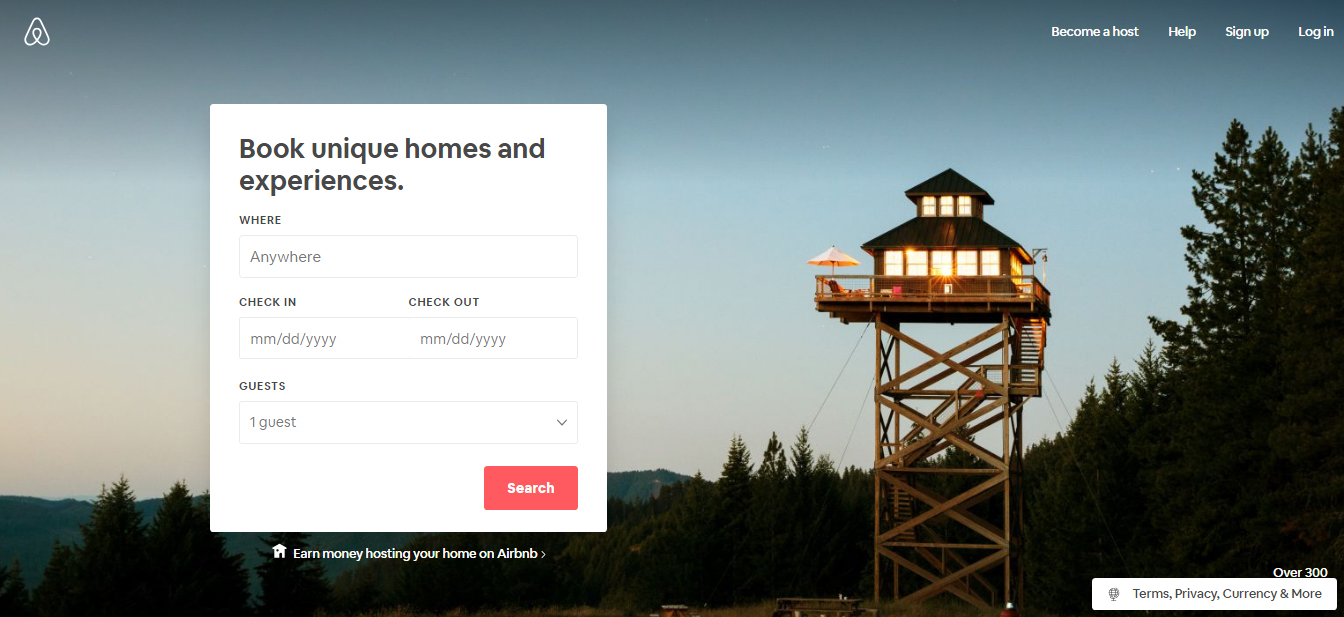Screenshot of the Airbnb website featuring its landing page. In the top left corner, the iconic Airbnb logo, resembling a white, flowery triangle or a boomerang, is prominently displayed. On the top right corner, there's a menu with options including "Become a Host," "Help," "Sign Up," and "Log In," all rendered in white font.

Dominating the page is a vibrant photo of a unique lodging option situated in a dense, wooded area. The structure appears to be a small house perched atop a tall wooden tower, evoking a treehouse vibe though it is not nestled within trees. The background shows a night sky with the silhouette of dense forests enhancing the secluded atmosphere of the accommodation.

Superimposed on the photo is a white box containing a search form. The form invites users to "Book unique homes and experiences" and contains fields labeled "Where," "Check in," "Check out," and "Guest." The placeholder text "Anywhere" hints at the flexibility of search locations. The guest dropdown is set to one guest by default. A conspicuous red search button sits at the bottom of the form, ready to initiate the search process.